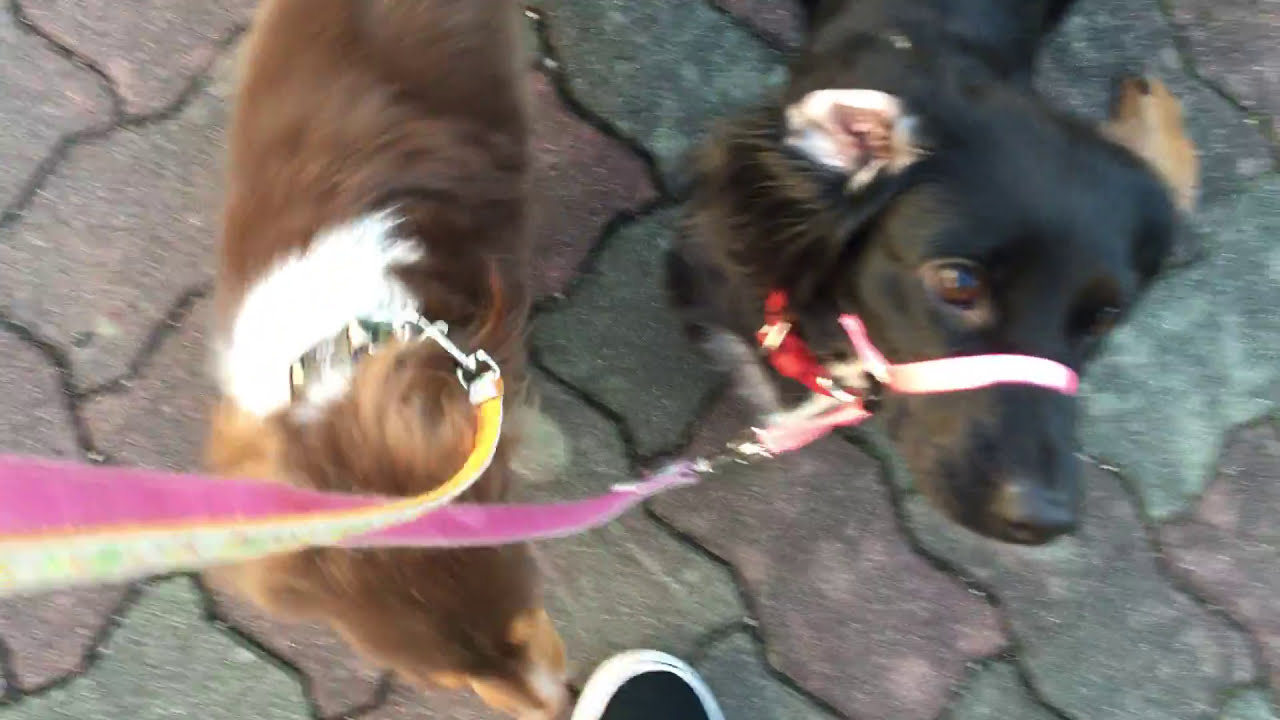The image captures a top-down view of two dogs walking on a brick sidewalk, probably taken by their owner. The picture is slightly blurry, suggesting the dogs are in motion. On the left, there is a mostly brown Border Collie with white patches around its neck and face, including a light tan stripe down its nose. This dog is attached with a white and gold leash. On the right, there is a black dog with long fur, wearing a red collar and a muzzle that secures around its nose. This dog has brown eyes, ears folded back so you can see inside the left one, and a pink leash is connected to its collar. In the bottom center of the image, a person's black shoe with white trim is visible, indicating the perspective of the photograph. The overall scene portrays the dogs as very furry and cute despite the slight out-of-focus quality of the image.